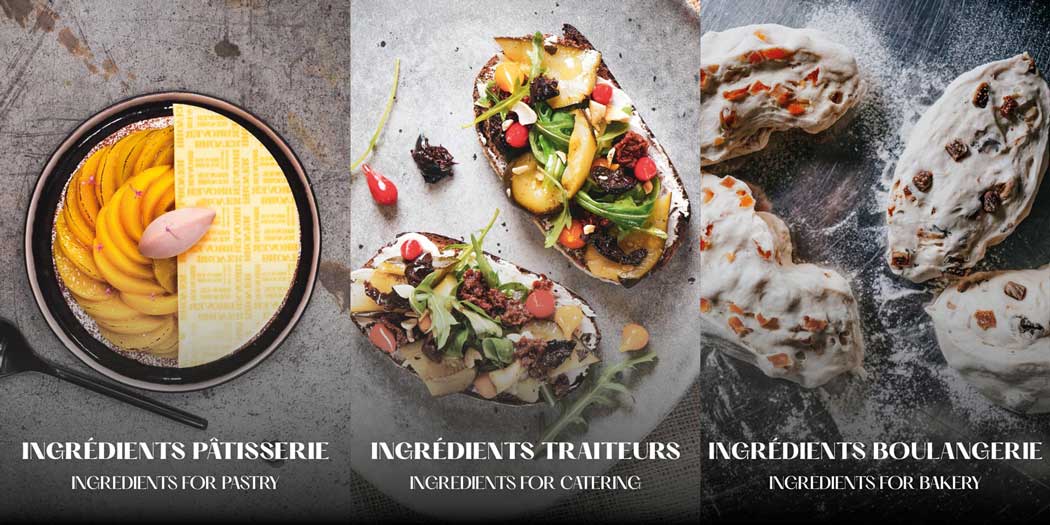The photograph is expertly divided into three equal sections, each showcasing a different culinary delight. The first section displays a sophisticated dish that features spiraled slices of what appears to be fruit or pastry, elegantly arranged on a circular black plate, accompanied by a black spoon. This dish, highlighted under the label "Ingredients for Pastry," includes a decorative half-circle element and a pink object at its center, adding to its visual appeal. The middle section, captioned "Ingredients for Catering," presents a vibrant spread of toast topped with a variety of fresh greens, vegetables, nuts, and possibly fruit. The final section, labeled "Ingredients for Bakery," features dense, white pastries adorned with a frosting and bits of dried fruit, set against a stone surface dusted with powdered sugar. The captions in French and English suggest these images are part of an advertisement for a restaurant, cooking class, or fresh ingredients, and the overall presentation is both colorful and appetizing.